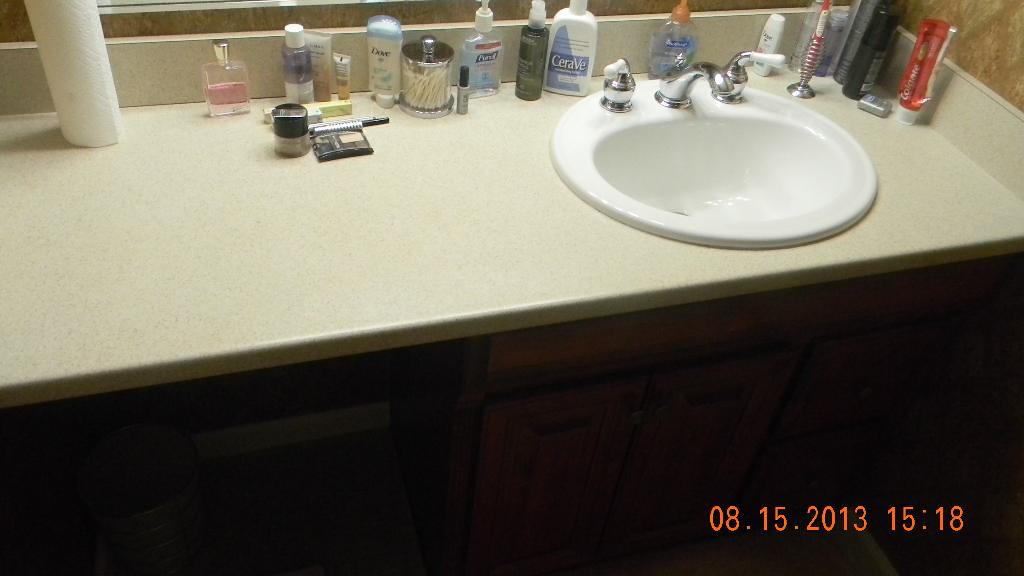Photograph of a bathroom sink with a yellowish, pale countertop. The sink is white and rounded, featuring sleek chrome fixtures. Above the countertop hangs a mirror. The cabinetry below is made of brown wood. The walls are adorned with a golden wallpaper design. On the far left side of the countertop, there is a roll of paper towels. Moving from left to right, one can see a bottle of perfume, assorted makeup items, deodorant, Q-tips, multiple bottles of lotion, hand soap behind the sink, a toothbrush, shampoo, body wash, toothpaste, and various bottles of hair products. The image has an orange time stamp at the bottom reading "08-15-2013" and "15:18".